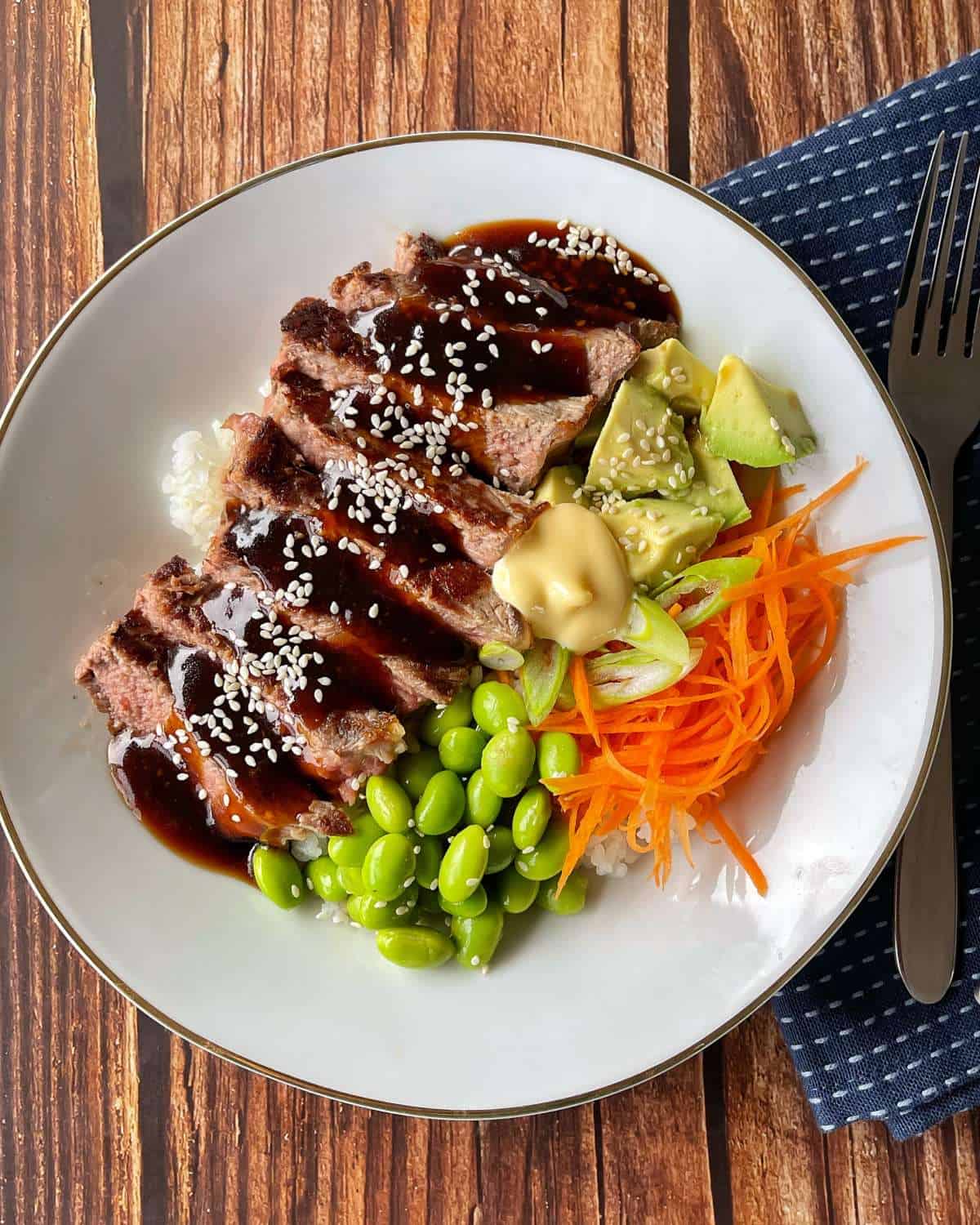In this overhead view of a dish, we observe a beautifully arranged meal on a circular white plate. The plate, which appears generally flat with a subtle dip in the center, features a variety of colorful ingredients positioned strategically around its face. On the left side of the plate, there are tender pieces of meat drizzled with a rich, dark brown sauce and garnished with a sprinkling of white sesame seeds. Moving rightward, a serving of vibrant green peas sits bathed in a light yellow sauce, adding a fresh and tangy contrast. Adjacent to the peas is a cluster of food with a lush green hue, possibly steamed vegetables or a dollop of leafy greens. Positioned at the bottom of the plate are strikingly bright orange carrot slices, providing a pop of color to the otherwise earthy palette.

Beside the plate on the right-hand side, there is a neatly placed blue napkin, with a silver fork resting vertically along its length. The dish is set on a brown table, whose warm tones serve as a backdrop, enhancing the overall presentation of the meal. This meticulously set arrangement invites an appreciation of both the visual appeal and the gastronomic experience.